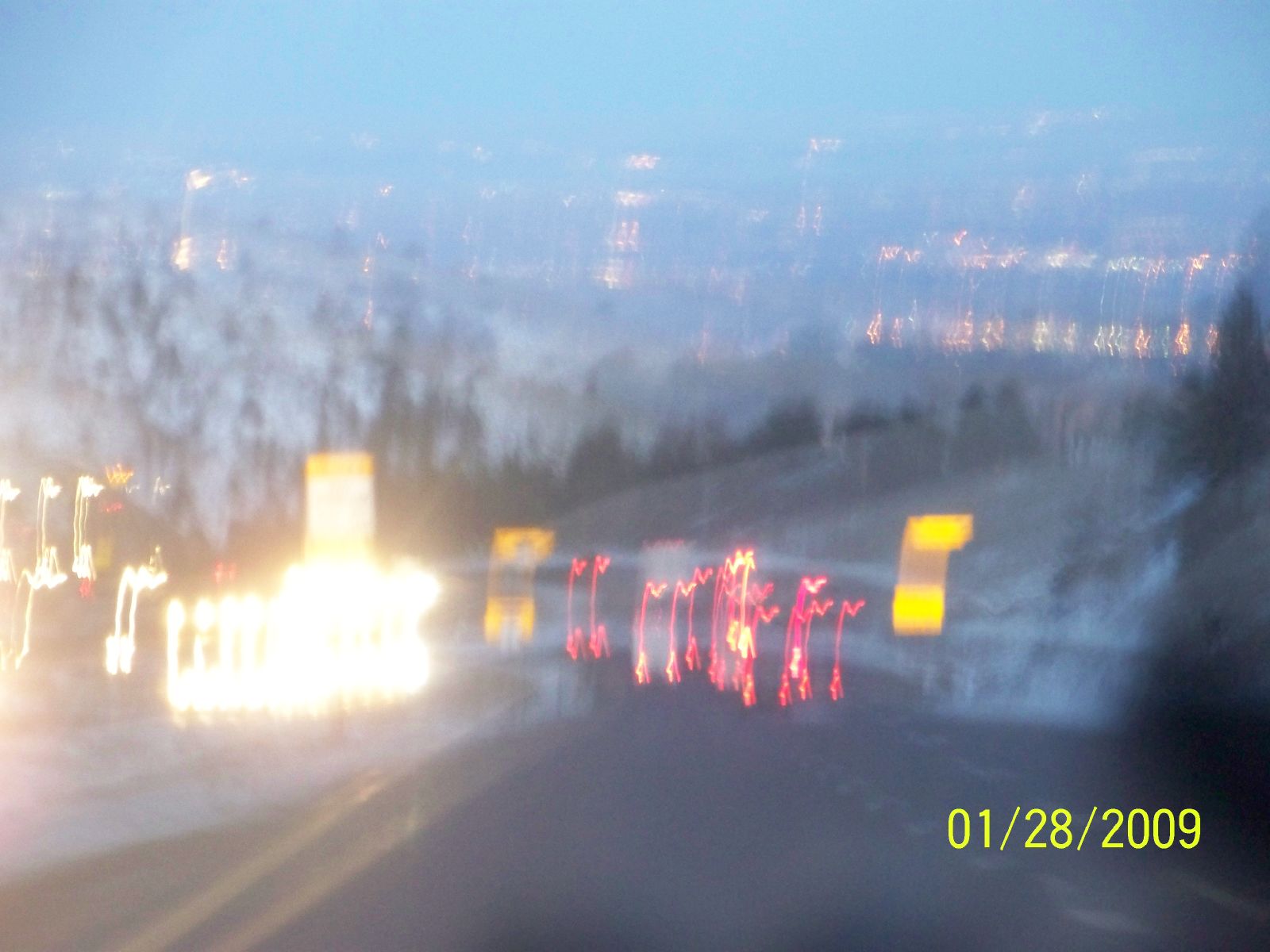Photographed from within a car, this image captures a winding road viewed through a windshield, adding an ethereal reflection that creates an intriguing optical illusion. The entire scene is enveloped in a dreamy, blurred quality, accentuated by the distorted glow of car headlights. The road, demarcated by yellow center lines, cuts through a snow-covered landscape. To the right, a small hill dusted with white rises up, leading to a majestic, snow-capped mountain adorned with numerous trees. In the background, a clear blue sky peeks through, partially obscured by the overlapping lights and reflections that lend a mystical aura to the photograph.